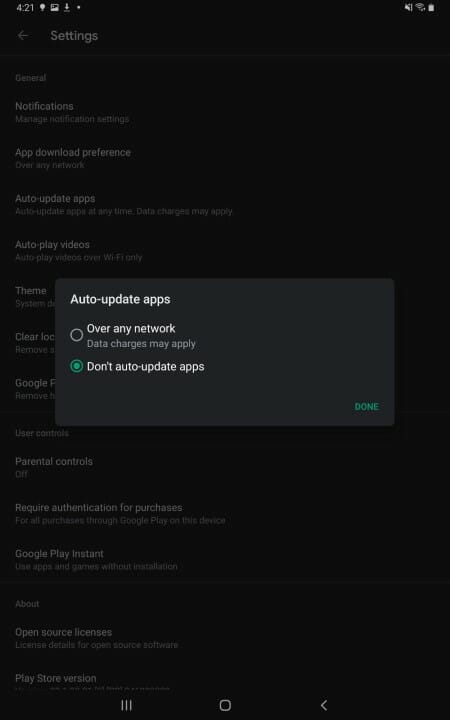The image depicts a mobile device's settings screen in dark mode. The background is a deep black, while a gray pop-up page is prominently featured in the center. This pop-up page displays white text detailing options under "Auto-update apps." Specifically, it provides options for auto-updating apps over any network (with data charges possibly applying) or not auto-updating apps, with the latter option checked off. A green "Done" button is situated at the bottom-right corner of the pop-up.

In the darker background behind this pop-up, the status bar is visible. The upper left corner shows the time as 4:21, alongside icons for a light bulb, indicative of active features or settings, and a download icon. The upper right corner displays connectivity icons, including a data or Wi-Fi signal and a battery level indicator. Below these, the word "Settings" is followed by a left-pointing arrow, indicating a back navigation option.

Further details below the primary options include "General," "Notifications," and "Message notification settings." Additional settings related to app management are also listed, such as "App download preference" (set to over any network), "Auto-update apps" (with an option for any time but currently disabled due to data charges), and "Auto-play videos" (configured to play only over Wi-Fi). Parental controls are noted as off, and authentication is required for all Google Play purchases on the device. Options for "Google Play Instant" allow the use of apps and games without installation, and "About" provides open source licenses and Play Store version information.